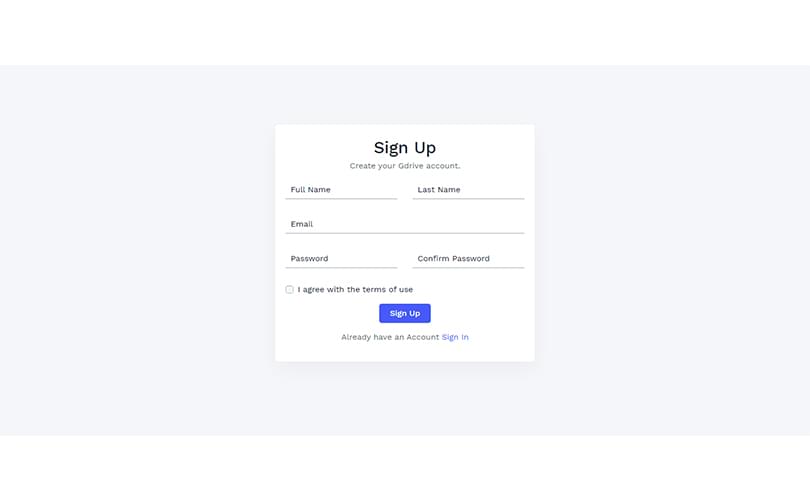Here is a detailed and cleaned-up descriptive caption based on the provided voice note:

---

The image features a user interface with a gray background. At the center, there is a prominent white box outlined in black. At the top of this box, bold black text reads, "Sign up." Below that, a subheading states, "Create your G Drive account."

The form begins with a line labeled "Full Name," accompanied underneath by an empty black bar for input. This is followed by a small gap and then an identical setup for "Last Name" with another input bar.

Next, you'll find a section for "Email Address," which has a longer input bar extending across the width of the form. Below this, there is a "Password" field followed by a similarly styled "Confirm Password" section.

Adjacent to these fields is an unchecked box with a label stating, "I agree with the terms of service."

At the bottom of the form, there's a blue button with white text that reads, "Sign up." Below this are smaller blue text links reading, "Already have an account? Sign in."

The overall design is minimalistic, focusing on ease of use for creating a new G Drive account.

---

This detailed caption encapsulates the interface's structure and visual elements more clearly and cohesively.